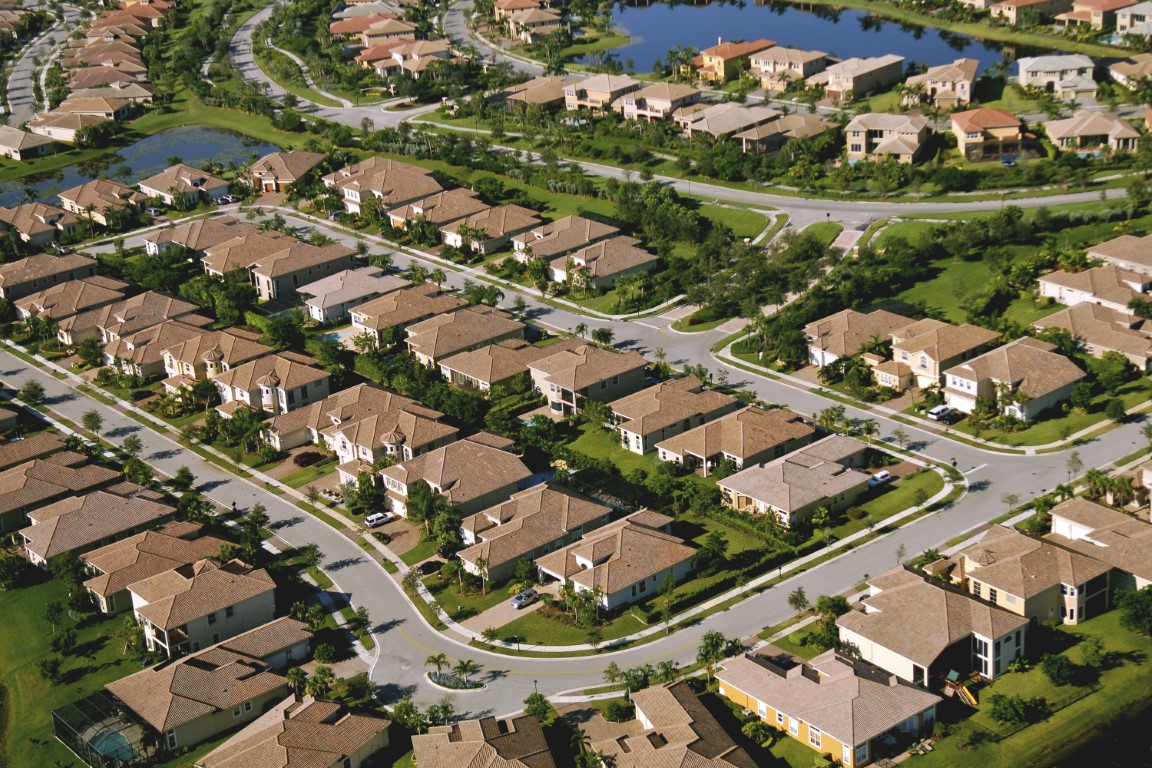The image depicts a well-organized, residential neighborhood from an overhead perspective during the day. The main section of the neighborhood forms a rectangular block of beige houses with brown tile roofs, divided by two mini roads that connect to a main road labeled as "C." These houses are aligned back-to-back, separated by narrow pathways, backyards, and a few green spaces. In this organized layout, most houses share similar architectural styles and roofing colors, though there is occasional variation such as a prominent yellow house on the right. 

In front of the houses, cars are parked along the streets lined with young trees, including palm trees, suggesting a recently developed area, likely in a place with a warm climate such as Florida. On the upper left side of the image, there is a small, possibly man-made lake separating the main rectangular section of houses from another housing section. Similarly, on the upper right, another larger lake is visible, with additional houses situated around it. Both lakes accentuate the community's aesthetics and could serve as recreational or drainage features. The overall image depicts a meticulously planned suburban development with interconnected streets, rows upon rows of uniformly styled homes, abundant young greenery, and multiple small bodies of water enhancing the neighborhood's scenic appeal.